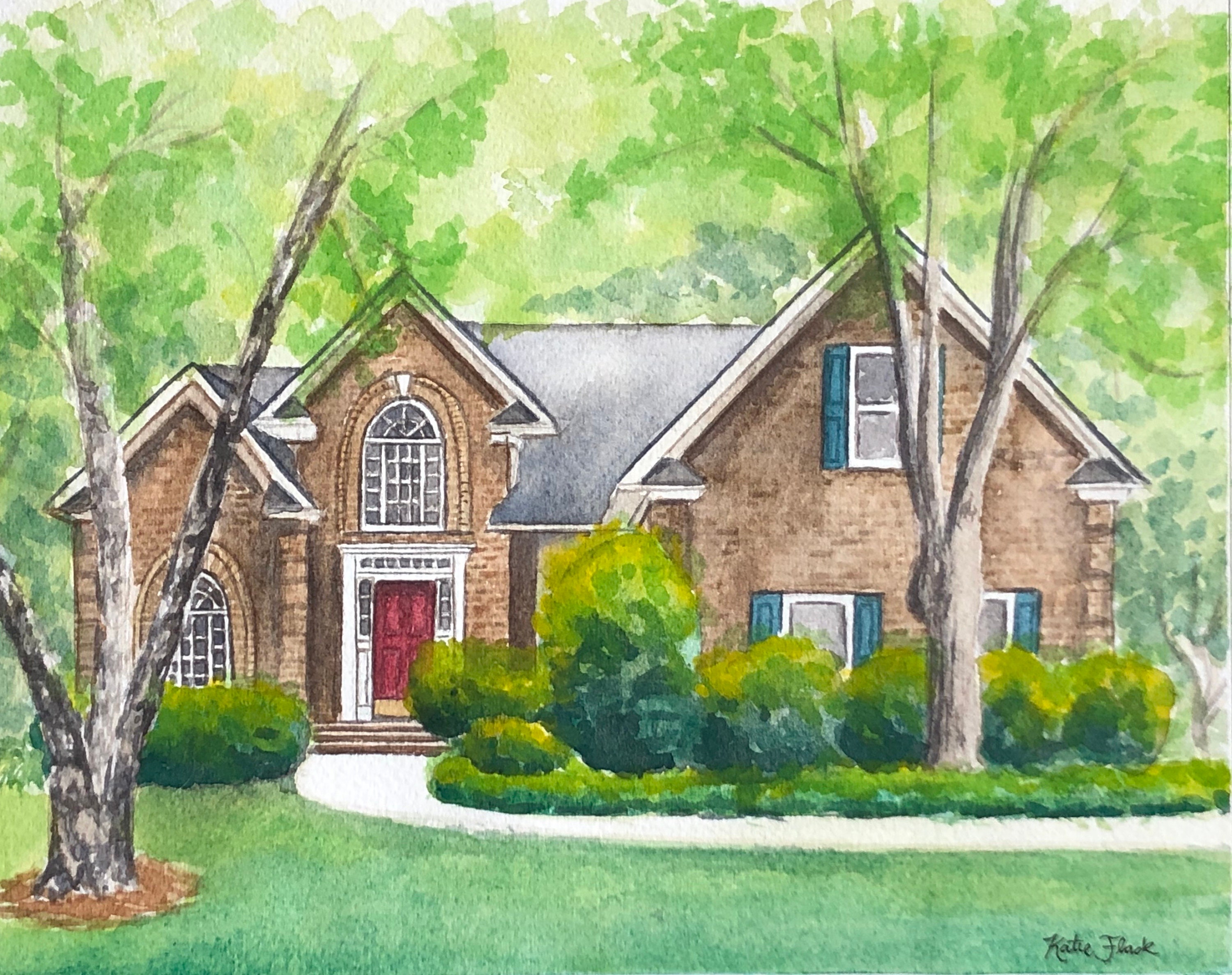This detailed watercolor painting by Katie Flass depicts a two-story brick house with a mansion-like appearance. The house features a complex, pointed roof structure highlighted in three distinct areas. The facade showcases a combination of red and brown bricks, adding depth and texture to the home. The central part of the house includes arched windows with elegant white frames that crisscross, topped by arched brick molding. Above the red wooden front door, framed in white with gold accents, there are three small window sections on either side near the top, allowing light to seep in. The door is accessible by three steps leading up from a curving walkway painted in white.

On the right side of the house, the white windows are accented with green shutters, while the left side of the house is distinguished by more artistic oval-shaped windows and additional arched brick molding. The left window also features a white crisscross frame. The roof is rendered in gray, complementing the overall color scheme.

In the foreground, two large trees with varying shades of green—including deep hunter green, lighter green, and yellow—frame the house. One tree stands to the left, planted with mulch around its base, while the other is positioned to the right. Between the trees and the house, the garden is filled with diverse shrubs in different sizes and shades of green. The lawn is depicted as lush green grass, adding to the tranquil, natural setting.

The entire scene is highly stylized, with leaves and foliage represented by splotches of green paint, creating a vibrant and lively ambiance. Notably, the painting omits any depiction of the sky, directing full attention to the richly detailed house and its surroundings. The artwork is signed by the artist, Katie Flass, cementing its authenticity and artistry.